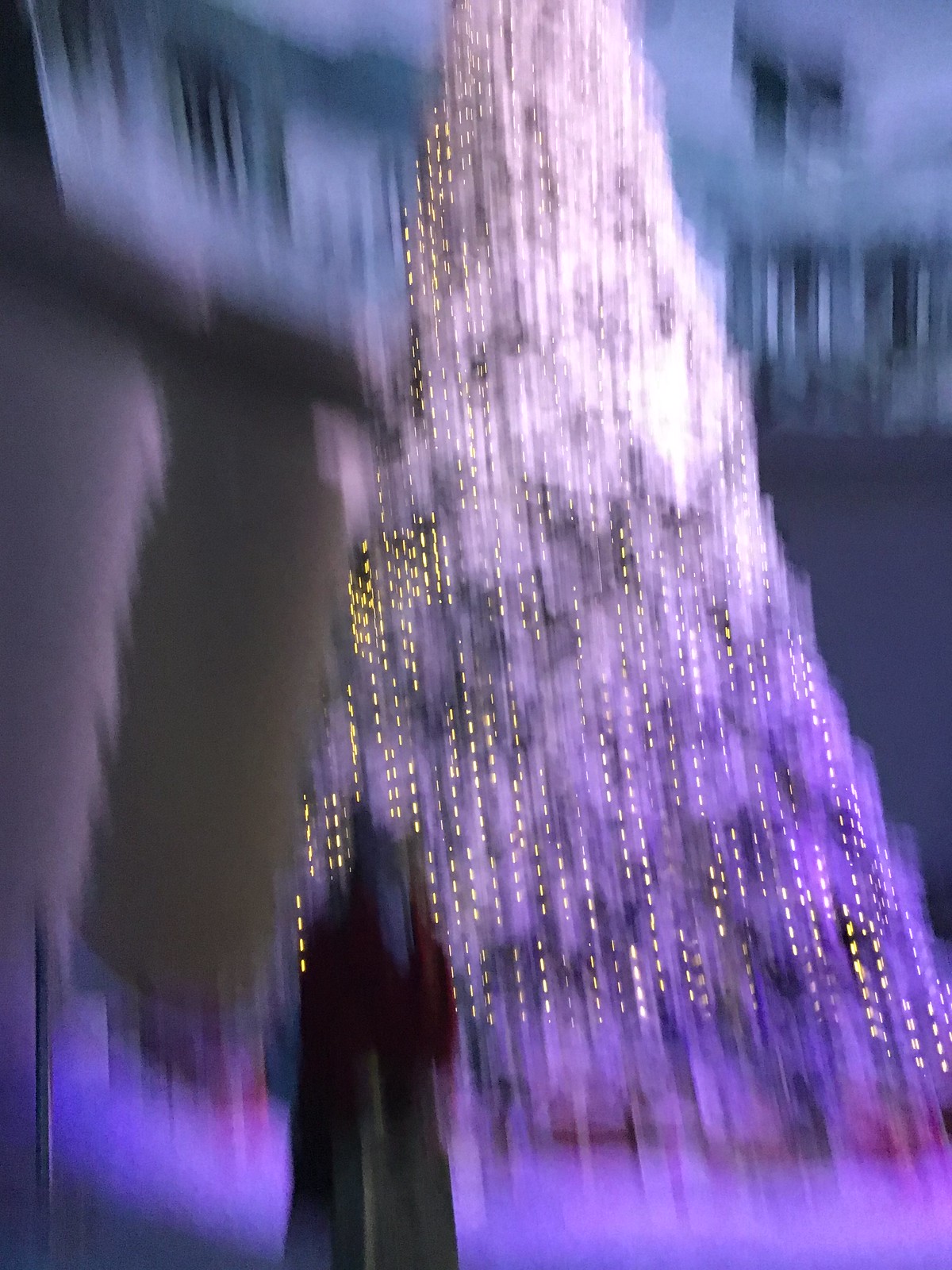The photograph is a very blurry, low-lit indoor image, likely taken during evening or nighttime with the camera moving vertically. In the foreground, there are two individuals, both wearing red shirts and possibly jeans or grayish-tan pants. One of the individuals might have a beard. Behind them, there's a large, tall Christmas tree that extends to a second-floor level, adorned with yellow or golden lights. The tree appears to be lavender in the blur, possibly snow-covered, giving it a soft white appearance at the base. The background features distorted, white-colored buildings in what looks like a rounded atrium with metal poles and ropes possibly blocking off the tree area. An overhead balcony or second tier is also visible.